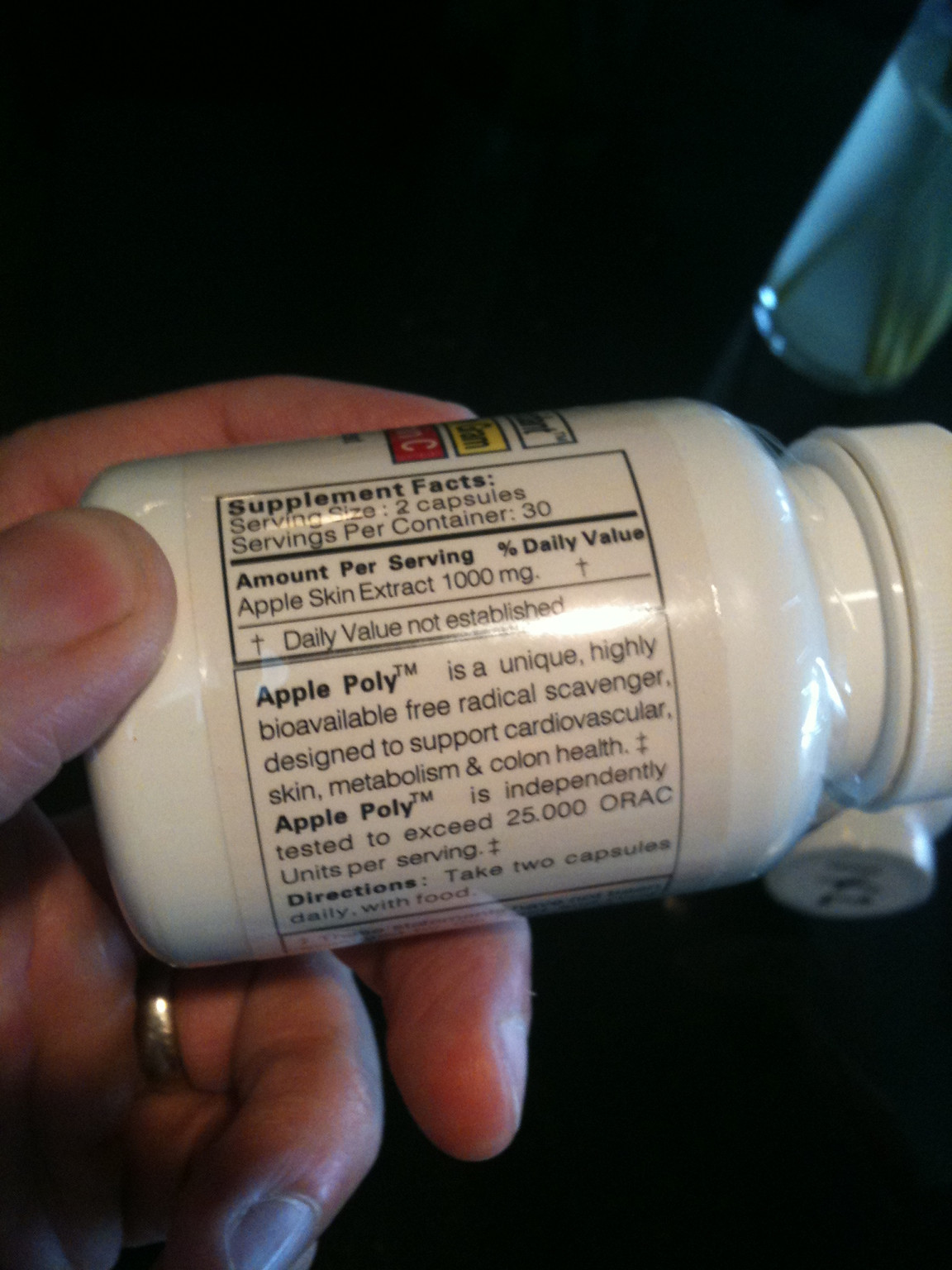The image depicts a close-up of a person's left hand holding a round, opaque white bottle with a white screw-top lid, against a dark, predominantly black background. The bottle is slightly horizontally positioned, with the cap on the right side of the frame and the bottom of the bottle resting in the individual's hand. The visible portion of the label focuses on the supplement facts, printed in black ink on a white background. Key details on the label reveal that the product is an over-the-counter supplement named Apple Polly™, which is a unique, highly bioavailable free radical scavenger designed to support cardiovascular, skin metabolism, and colon health. Each serving size is two capsules, with 30 servings per container. The amount per serving includes 1,000 milligrams of apple skin extract, providing over 25,000 ORAC units per serving. The directions instruct users to take two capsules daily with food. In the upper right-hand corner of the image, a small blue item is visible but not clearly identifiable.